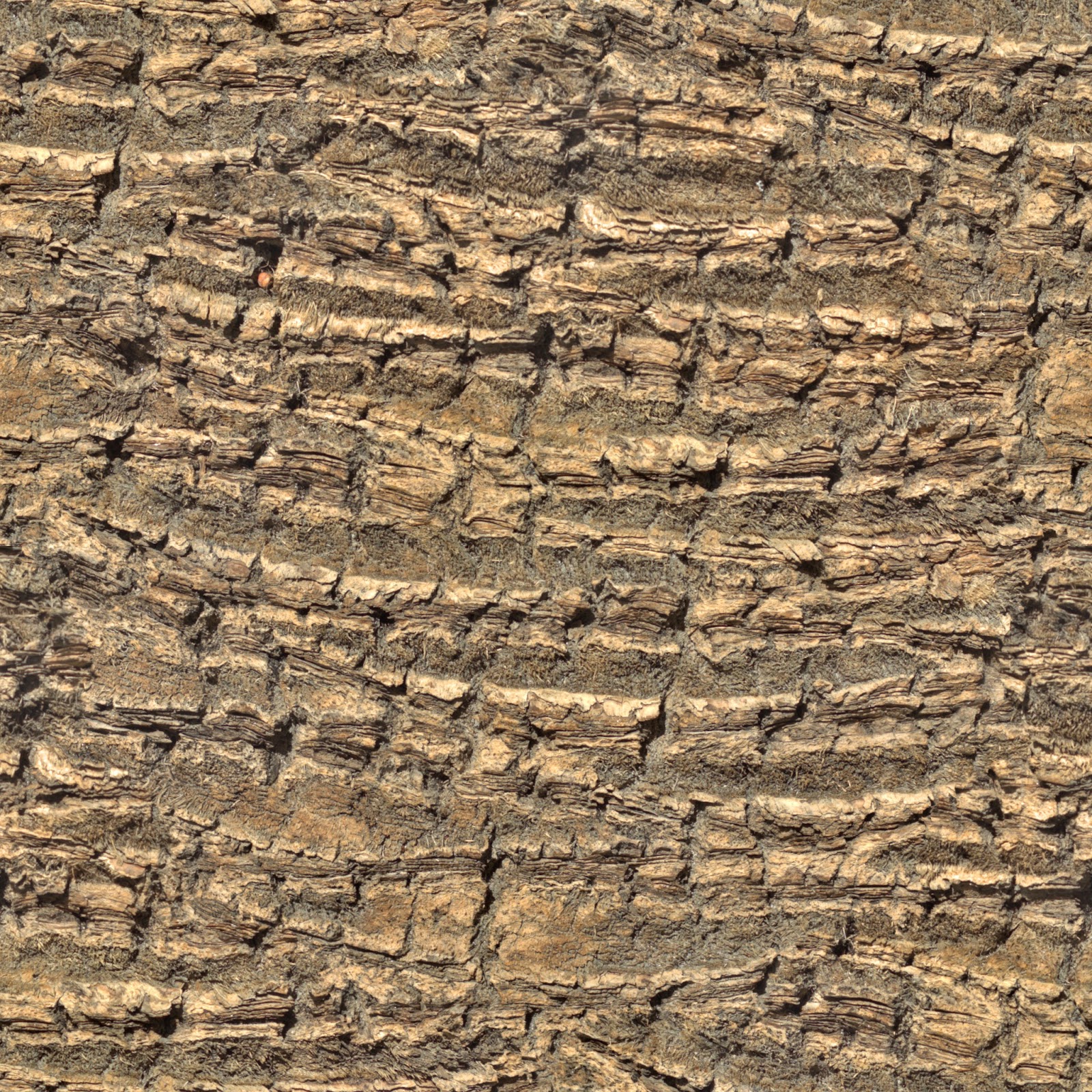The image depicts a vast and rugged rocky formation, potentially resembling a mountain side or an expanse within the Grand Canyon. The scene is dominated by earth tones, primarily various shades of brown, black, and some streaks of white. The surface is highly textured, featuring numerous jagged, horizontal striations and divots that give the appearance of a massive, weather-beaten wall. These rocky segments create a complex pattern of raised edges and recessed areas, reminiscent of a drought-stricken, cracked landscape. There is a notable absence of vegetation, emphasizing the barren, dehydrated nature of the terrain. Interspersed among the rocky surface are small holes and crevices, one of which contains a mysterious, small orange object, too indistinct to identify. The entire formation, despite its rough and uneven texture, is well-lit, casting a clear, bronzy sheen across the image.